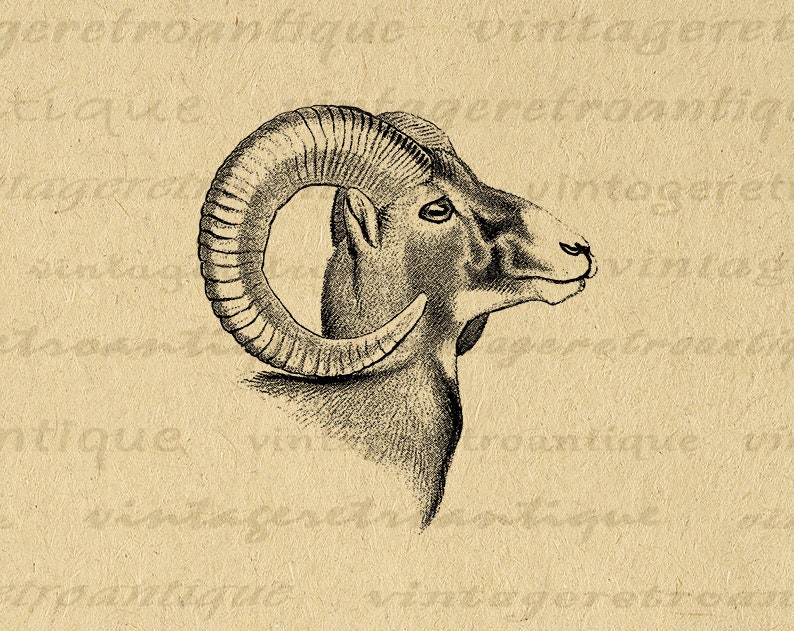The image depicts a rectangular, six-by-four-inch artwork featuring a detailed pencil drawing of a ram's head in side profile. The background is a light tan, reminiscent of lighter-colored brown paper, and is overlaid with various words in a watermark style. These words, written in both print and cursive, appear in a shade slightly darker than the background and include "RETRA ANTIQUE" and "Vinta Garrett" among others, repeating subtly across the paper. The ram, shown in a black or dark pencil, features thick, curled horns extending from just above its ears, wrapping around to below its cheek. The ram's prominent details include its closed mouth, a white nose, and white under its neck, contrasting with the darker pencil shading used for the rest of its head.